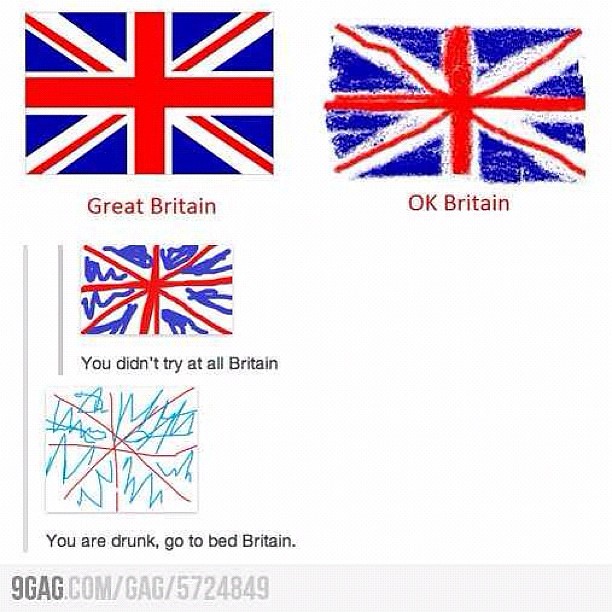The image from 9gag.com features a humorous depiction of the British flag's progressive distortion through four versions. The top-left corner displays a clear and sharp computer-generated Union Jack labeled "Great Britain," with precise red, white, and blue colors. Adjacent to it in the top-right, a slightly faded and wavy hand-drawn version is labeled "OK Britain." Beneath the sharp flag, another flag is crudely drawn with ink pens or markers, significantly distorted and humorously captioned "you didn't try at all, Britain." At the bottom of the image, a nearly unrecognizable flag, scribbled with blue and black pens on a white background, is hilariously captioned "you are drunk, go to bed, Britain." The overall comedic progression illustrates the declining quality of the British flag in tandem with the captions, emphasizing the state of mind humor. The image is tagged with the source 9GAG.com/gag/5724849.